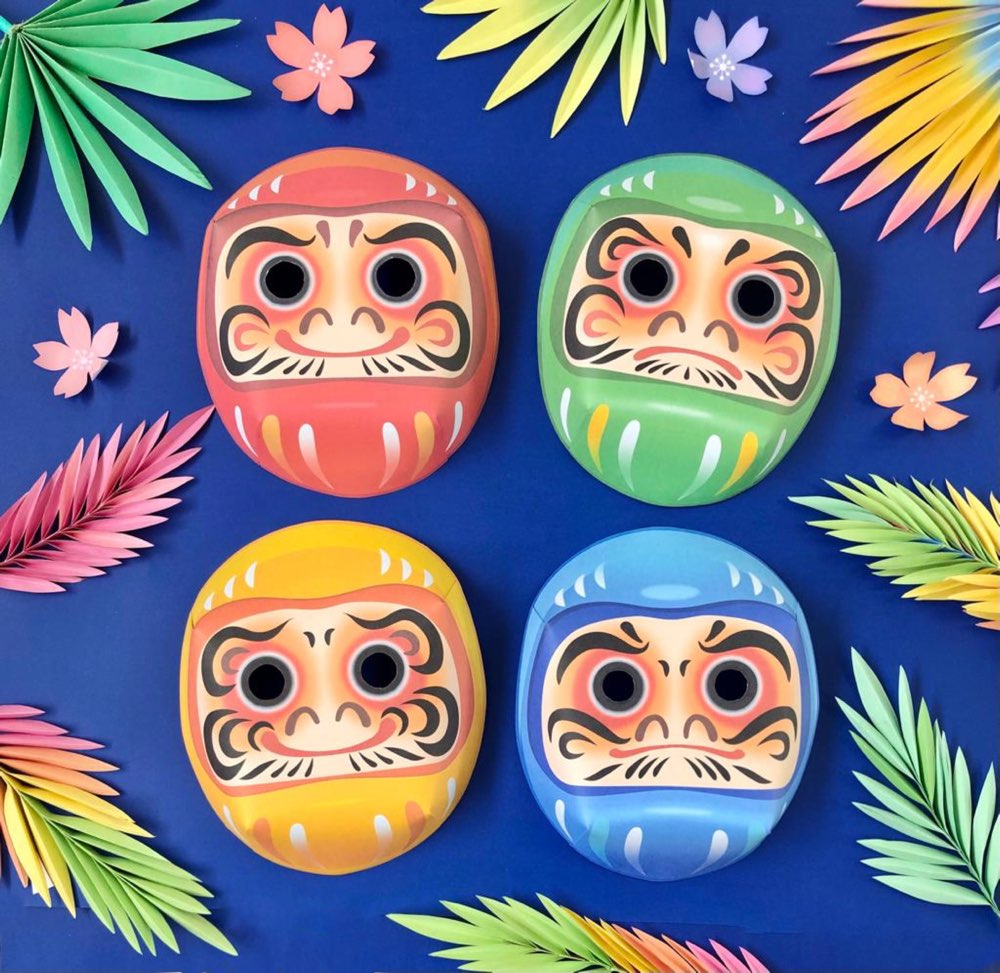The image features a vivid royal blue background adorned with an array of colorful leaves in shades of green, pink, yellow, orange, and blue, scattered around the edges. At the center, four cartoonish, oval-shaped masks are arranged in two rows, each with distinct expressions and vibrant colors. The top-left mask is red with black eyebrows, black eyes encircled by white and red rings, a glossy peach complexion, and a red smile. To its right, the green mask mirrors the same facial features but sports a frowning expression. Below, the left mask is yellow with a neutral look, and the right blue mask has a similar neutral or slightly frowning demeanor. The central faces are highlighted with peach tones and gray accents, giving them a glossy, animated appearance, reminiscent of computer-generated artwork.